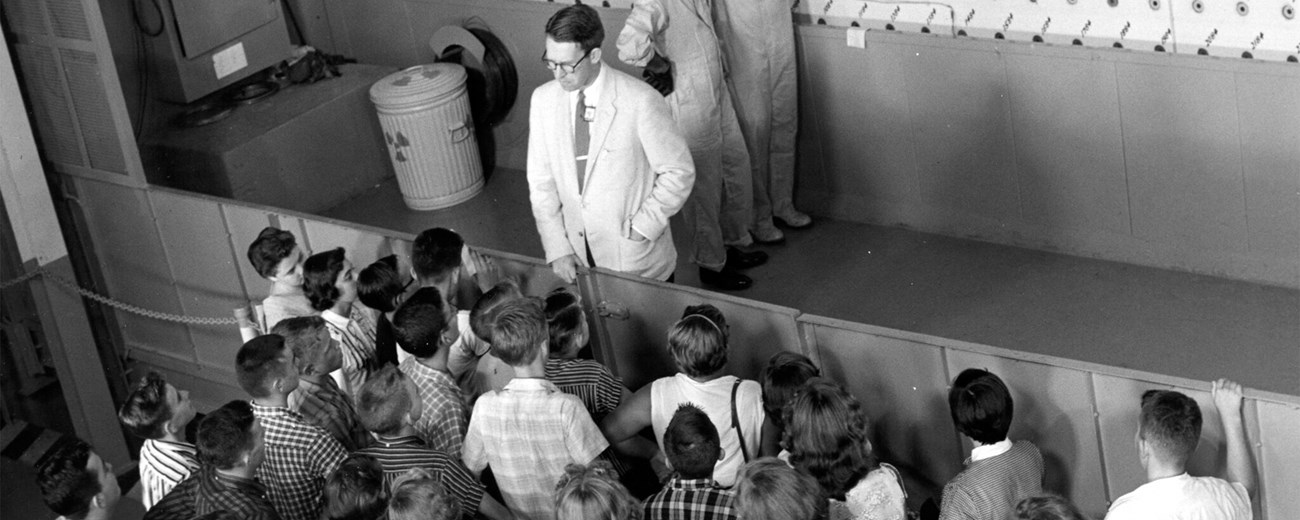This black-and-white photograph captures a group of children on a school field trip, observing a scientist at work. The scene is framed by a waist-high wooden or metal wall that separates the children from the scientist. The central figure, a man dressed in a white suit with a tie and glasses, exudes an air of authority and engagement. He stands right in front of the wall, with one hand in his jacket pocket and the other resting on the wall, as he addresses the children gathered before him. In the background, against the far corner, there's a white metal garbage can marked with a biohazard symbol, hinting at a laboratory setting. Two other men, clad in white jumpsuits and gloves, stand side-by-side, though their heads are cropped out of the frame. The children are clearly captivated, their faces turned toward the scientist, absorbing the lesson from a safe distance.